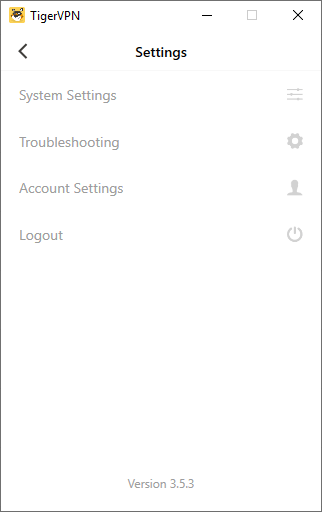Here is a cleaned-up and detailed caption for the image:

"The screenshot displays the settings area of the Tiger VPN app. At the top-left corner, the Tiger VPN logo is prominently visible. On the top-right corner, there are three standard window control buttons: minimize, restore down, and close. Centered below the top bar, the word 'Settings' is clearly marked with a left-pointing arrow to its left, suggesting a navigation option to go back.

The settings menu is organized with gray-colored options, each accompanied by a matching icon. The options listed are:
1. System Settings
2. Troubleshooting
3. Account Settings
4. Logout

At the very bottom of the page, the app version is noted as 'Version 3.5.3.'"